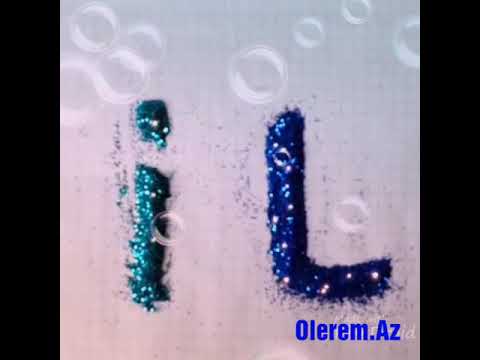The image resembles an album cover or an advertisement. It features two black vertical lines on each side, framing a central rectangular area with an ombre background that transitions from light purple to a blush pink. The top of the background has a circular, bubble-like pattern. In the middle, there's a lowercase 'i' made of teal glitter and a capitalized 'L' in blue glitter, both prominently displayed. Below the letter 'L', the text "OLELEM.AZ" is written in bold blue letters. A bubble appears above the 'i', adding to the decorative elements in the background.